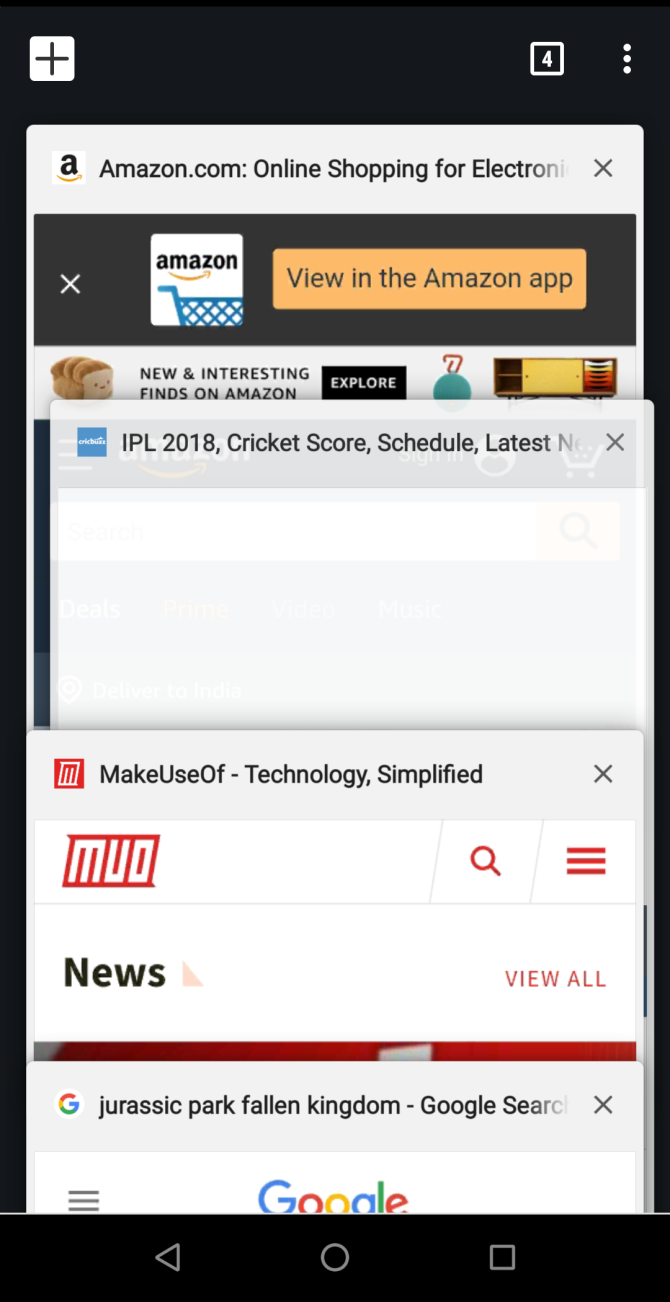The image displays an Amazon page as viewed on a cell phone, featuring a primarily black background with several focal points and overlays. At the top left corner, there is a white square with a red cross inside, while the top right corner has a bordered white box containing the number four and three vertical dots beside it. Ironically, the next visual element is a prominent white rectangle set against the black background. Inside this rectangle is the Amazon logo — a stylized 'a' with a swoosh underneath — and text that reads, "amazon.com: online shopping for" followed by "e-l-e-c-t-r-o-n-i," which fades out before completing the word.

Below this, another black rectangle appears, holding a white 'X' on the left side and an Amazon shopping cart icon. Adjacent to these icons is an orange button labeled "View in the Amazon app." The next section features a white card displaying the text "IPL 2018, cricket score, schedule, latest," which fades out with an 'X' towards the end.

Following that is another white card containing the text, "Make use of - technology, simplified." The final card shows the Google logo with the text, "Jurassic Park Fallen Kingdom - Google search," which also fades off after the letter 'C.'

At the bottom of the screen, there are three horizontal lines indicating a menu, and to the right of these lines sits the colorful Google logo.